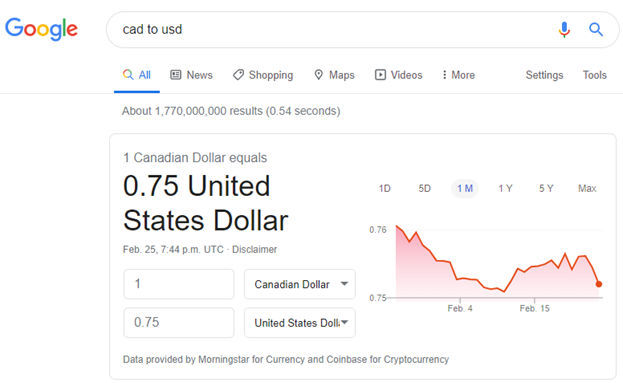The image depicts a Google search results page, specifically searching for "CAD to USD." The familiar Google logo is positioned on the left side of the search bar, while a microphone icon and a magnifying glass icon are located on the right. Below the search bar, various tabs like "All," "News," "Shopping," "Math," "Videos," and "More" are displayed, with "All" highlighted in blue and underscored by a blue line. The search results reveal that approximately 1,770,000,000 results were generated in just 0.54 seconds.

A white box with a light gray outline on all sides prominently appears beneath these tabs. Inside, it indicates that "One Canadian Dollar equals 0.75 United States Dollars," timestamped at "February 25th, 7:44 p.m. UTC, with a disclaimer." This box contains a text field that reads "1," next to a drop-down menu labeled "Canadian Dollar," followed by another text field that reads "0.75" adjacent to a drop-down menu labeled "United States Dollar."

To the right of this box is a graph that displays conversion trends over various periods, ranging from "1 day" to "5 years," with an additional "Max" option in the upper-right corner. The vertical axis on the left side of the graph ranges from "0.75" to "0.76," providing a visual representation of the currency conversion rate.